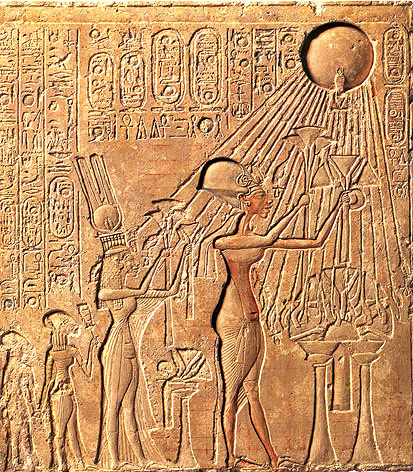The image is a detailed depiction of an ancient stone tablet, possibly originating from an Egyptian context, with intricate carvings that appear modern but retain an authentic feel. The scene illustrates a ceremonial gathering under a prominent circular figure, likely the sun, emitting rays toward several figures in the foreground. These figures, which include a queen and her subjects, are shown holding up glasses or staves, seemingly attempting to catch the sun's rays. The stone, of a sand or brown hue, suggests it was found in a desert setting. Surrounding the central image are hieroglyphs, structured both vertically and horizontally, further enhancing the artifact's ancient appearance. Despite its old-fashioned, etched-in design, the tablet's vibrant orange and yellow tones and the high quality of the image make the artwork vividly detailed.